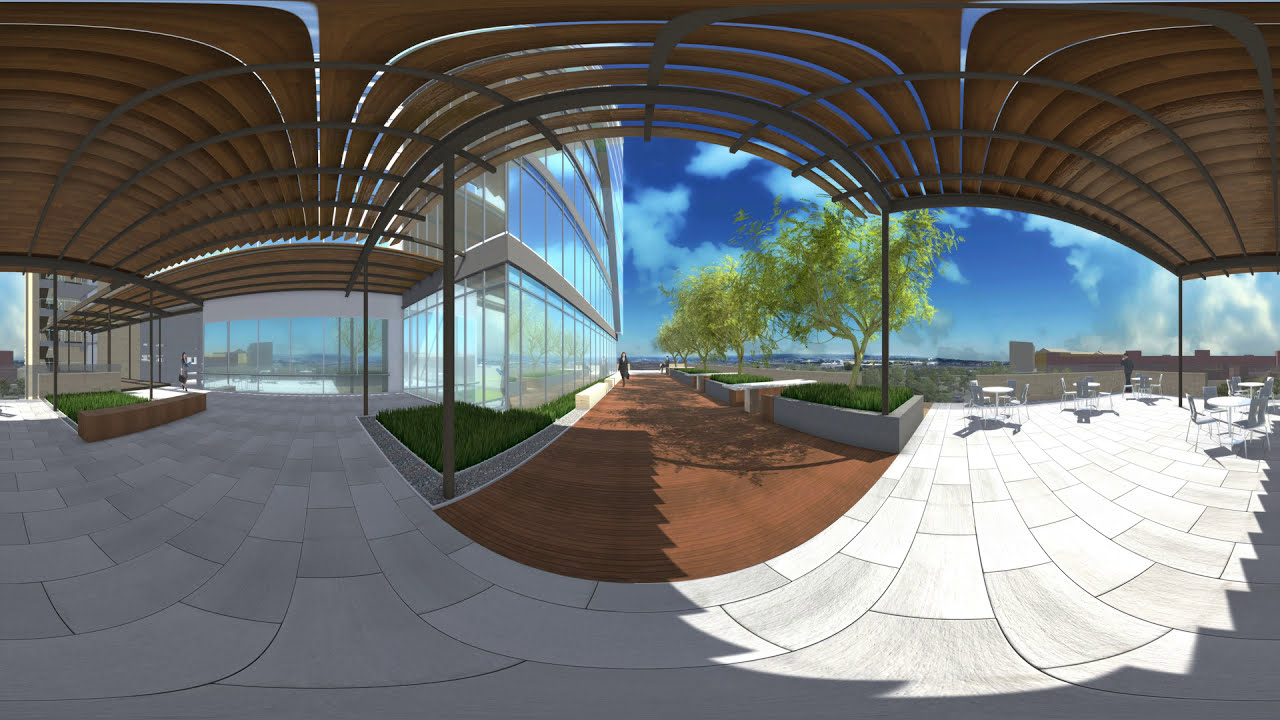The image portrays a surreal pavilion area that exudes elegance and modernity, possibly serving as a relaxing outdoor space for a hotel or fancy building. The ground is covered with large, light gray tiles forming a clean and official look. At the top, the pavilion features a large, brown slated roof with a distinctive series of arches and black stripes running across them. The focal point of the background is a triangular-shaped building made of glass and steel with many tall, reflective windows.

The pavilion is divided into three segments, each with planters containing grass and light-colored leafy trees. One segment has a brown path with a rounded edge where a single person walks straight ahead. To the right, there is a patio area outfitted with multiple white tables and chairs, inviting people to sit and enjoy a leisurely coffee break. The sky above is clear blue with scattering white clouds, further enhancing the serene ambiance of the scene.